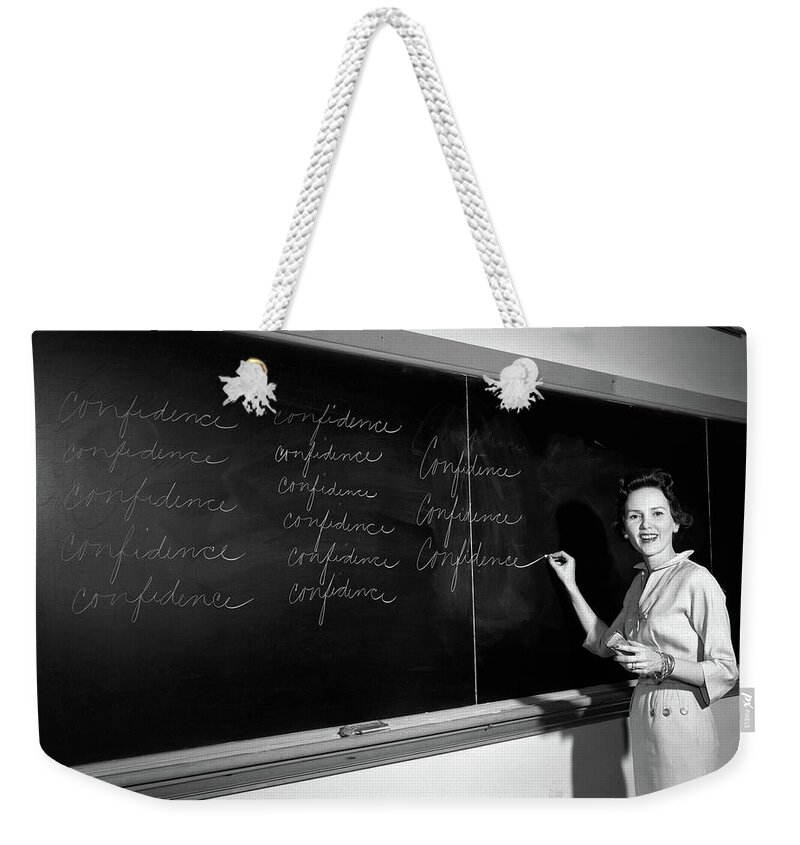In this detailed black-and-white image, which is displayed to look as if it is hanging by a cord against a white wall, a woman dressed in a work suit dress stands on the right side of the frame, facing the camera with a warm smile. The woman, likely from the 1950s or early 1960s, has short brunette hair and is adorned with bangles on her wrist and multiple rings on her fingers. She holds a piece of chalk and is captured in the act of writing the word “confidence” for the 15th time across several panels of a large chalkboard. The completed rows and the long tail on the final 'e' of the last word emphasize her diligent repetition. An eraser rests in a tray that runs the length of the board, and she also holds another eraser in her hand. The distinct vintage style and the meticulous detail in her writing suggest her role as a dedicated educator.